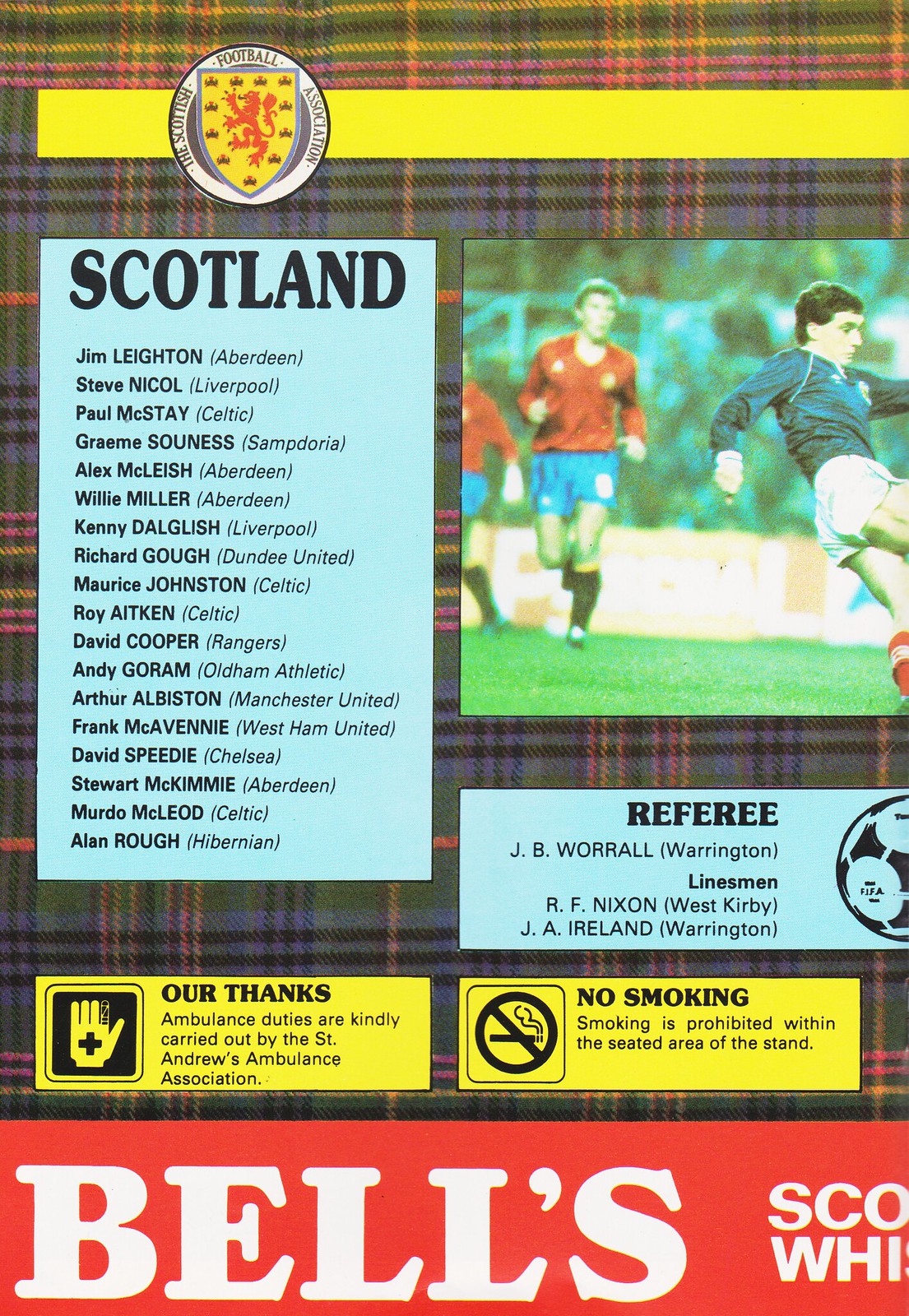The cover of the soccer game program features a distinctive Scottish plaid background reminiscent of a kilt. At the top, a yellow bar highlights the logo of the Scottish Football Association, which includes a shield with a lion. To the right, a vibrant photograph depicts soccer players in action: one player in a blue jersey kicks the ball while two others in red jerseys appear in the background. On the left, a blue text box titled "Scotland" lists the names of the players, including Jim Leighton (Aberdeen), Steve Nicol (Liverpool), Paul McStay (Celtic), Graeme Souness (Sampdoria), Alex McLeish (Aberdeen), Willie Miller (Aberdeen), Kenny Dalglish (Liverpool), Richard Gough (Dundee United), Maurice Johnston (Celtic), Roy Aitken (Celtic), Davie Cooper (Rangers), Andy Goram (Oldham Athletic), Arthur Albiston (Manchester United), Frank McAvennie (West Ham United), David Speedie (Chelsea), Stewart McKimmie (Aberdeen), Murdo MacLeod (Celtic), and Alan Rough (Hibernian). The list also includes match officials: referee JB Worrall (Warrington) and linesmen RF Nixon (West Kirby) and JA Ireland (Warrington).

Additionally, there are two notices in yellow at the bottom of the page. One expresses thanks to the St. Andrews Ambulance Association for providing ambulance services, accompanied by an illustration of a hand with a red cross and a bandaged finger. The other notice emphasizes that smoking is prohibited within the seated area of the stand. The bottom of the page features a red banner partially reading "Bells," likely referring to Bell's Scotch Whisky.